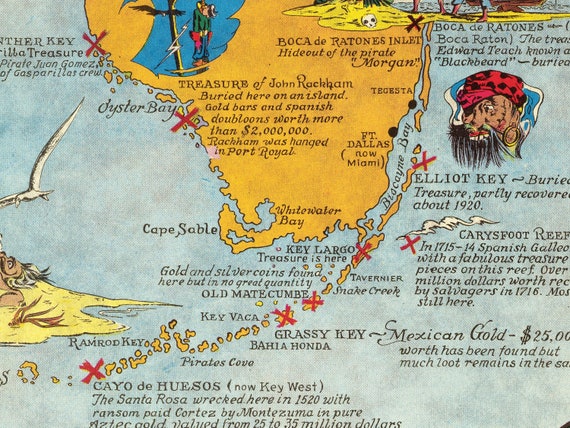The image is a detailed, humorous, hand-drawn treasure map that is wider than it is tall, resembling a pirate's map. The background of the map is blue, with a country depicted in a darker yellow hue. Scattered across the map are several small, intricate drawings and red X's marking supposed treasure locations. Dominating the right side is a sketch of a scraggly-bearded pirate, reminiscent of Blackbeard, adorned with a red cap with black spots, an eye patch, a peculiar mustache, and a large round earring.

Text on the map denotes various locations and clues related to pirate lore and hidden treasures. Notable mentions include "Treasure of John Rockman buried here on the island," "Gold bars and Spanish doubloons worth more than two million," and historical references like "Rockham was hanged in Port Royal." The map highlights geographical features and locales such as Cape Sable, Key Largo, Pirate's Cove, Grassy Key, Bahia Honda, and Oyster Bay, along with other spots like Elliott Key which notes "buried treasure, partly recovered about 1920," and Carey's Foot Reef with mentions of Mexican gold worth $25,000, yet to be fully recovered. Additional marked sites include Fort Dallas, Boca Raton Inlet, and Cayo de Husos, now known as Key West.

Overall, the map appears to be a whimsical depiction of pirate mythology with a wealth of small text and details, crafting a rich narrative of hidden treasures scattered across an island landscape.